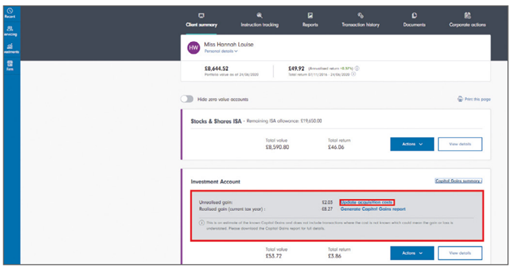This is a detailed caption for an image:

"A blurry screenshot taken from a financial website, likely a desktop interface, showcases the online banking dashboard of an individual named Miss Hannah Louise. The page includes several sections displaying various financial products and amounts. The main balance visible reads £8,644.52 (currency somewhat unclear), accompanied by another figure, possibly £49.92. Further down, distinct sections are labeled 'Stocks and Shares ISA' and 'Investment Account,' each displaying separate, albeit unreadable, monetary amounts. The interface appears to consolidate Miss Hannah Louise's financial products on a single platform, but due to the small and blurred nature of the image, finer details remain indiscernible."